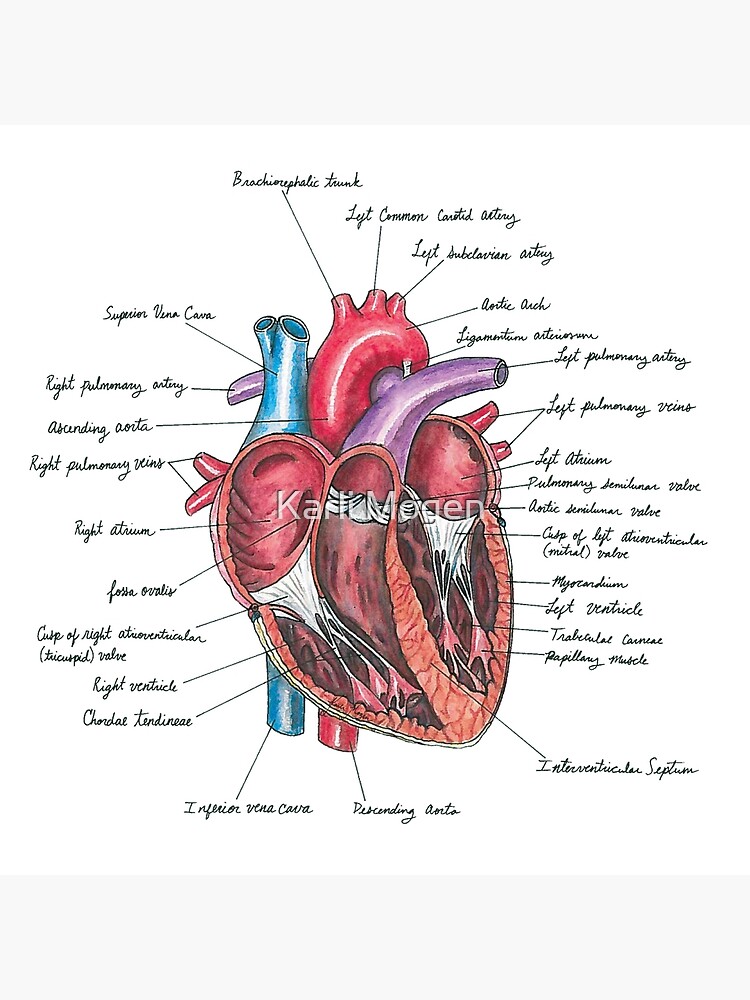This image is a detailed, hand-drawn, cross-sectional diagram of a human heart set against a white backdrop. There are thin light gray bars at the top and bottom, framing the main illustration. The heart is sliced in half, revealing its internal structures. Various parts, arteries, and veins are meticulously labeled with black cursive text. Each label is connected to its corresponding heart part by black pointer lines. The color palette includes reds, purples, blues, tans, and whites. Key features such as the aorta, left common carotid artery, left subclavian artery, aortic arch, left pulmonary artery, left pulmonary veins, descending aorta, and papillary muscles are distinctly marked. The image also highlights the atriums (right and left), the vena cava, the ventricles, and other anatomical details, each vividly illustrated in complementary colors, such as blue for the heart, red for the aorta, and purples and oranges for other veins and internal structures. This informative drawing provides a comprehensive visual guide to the heart's anatomy, with over 25 labeled parts surrounding it.